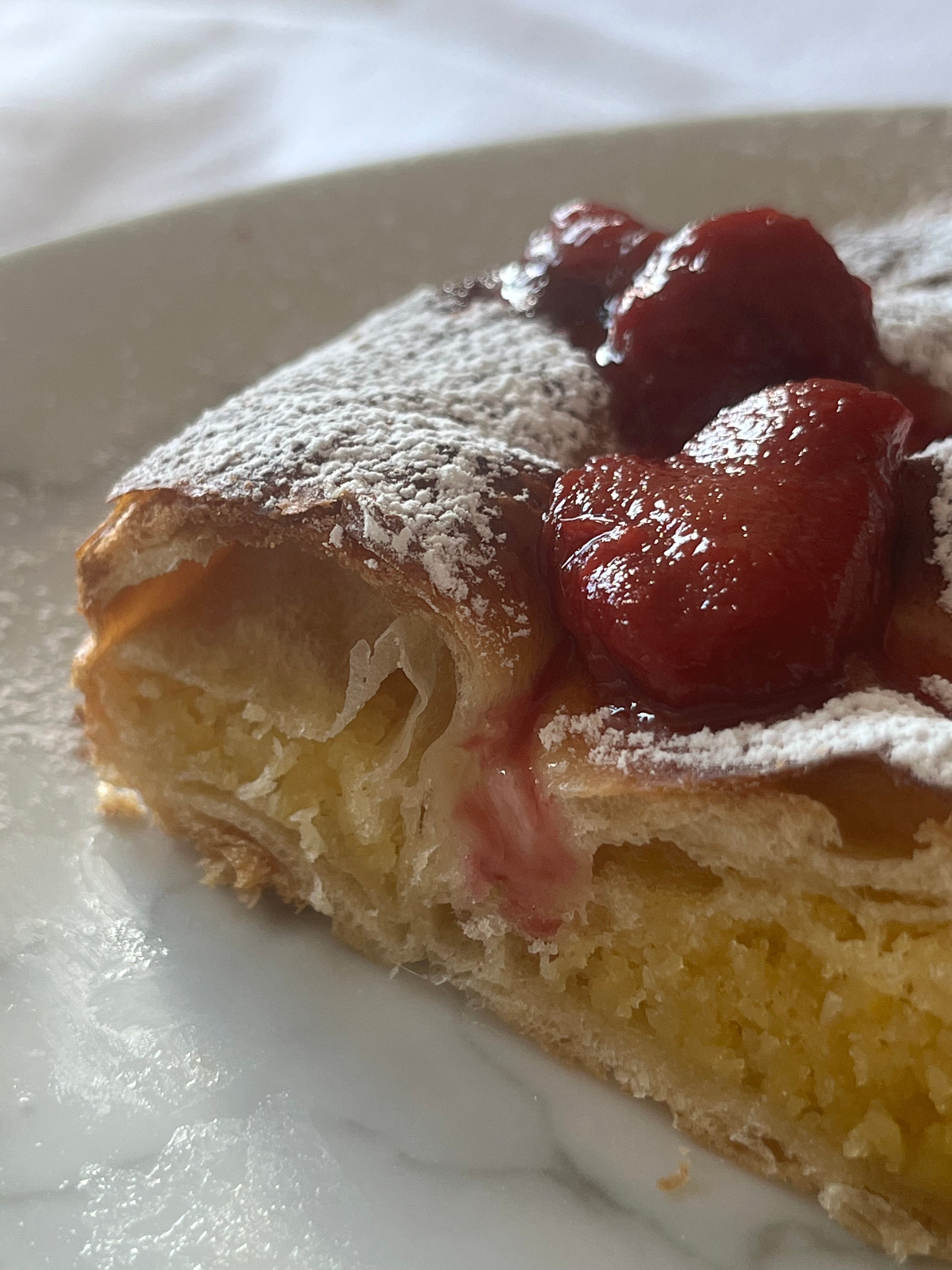The photograph is a vertically rectangular, full-color, staged indoor shot, possibly illuminated by natural or artificial light. The background is blurred but appears to be a white tablecloth with some light shining in from the upper left. The main focus is a slice of pie placed on a plain white plate. The pie features a yellow, cake-like filling encased in a flaky, brown crust, possibly phyllo dough, and is dusted with powdered sugar. On top of the pie are glossy strawberries and a red sauce, possibly mixed with cream. The detailed close-up captures the pie's deliciously crunchy exterior and appetizing interior.